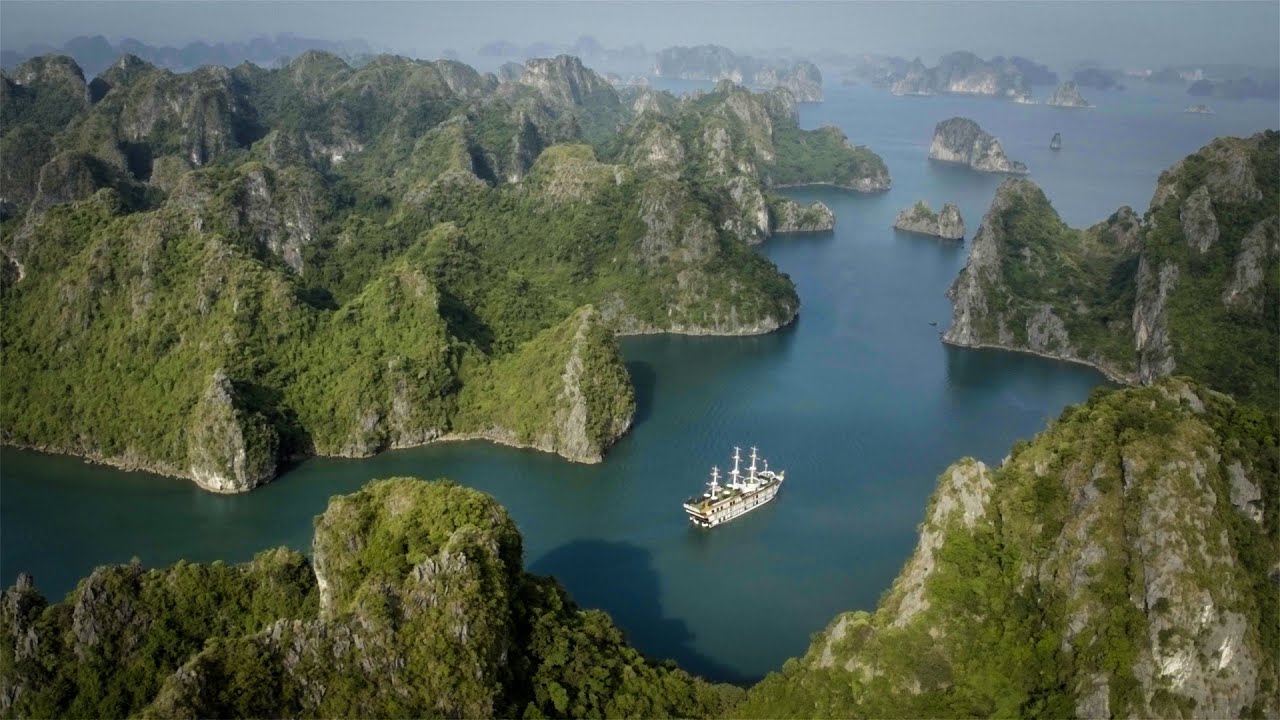The photo appears to be taken from a high vantage point, possibly from a drone, airplane, or helicopter, capturing a sweeping view of a winding fjord or river cutting through a mountainous region. The sky above is light blue with a touch of fog and mist, creating a somewhat obscured and ethereal background. 

Dominating the scene are steep, rocky cliffs and mountainous islands covered in lush green vegetation, with patches of gray rock peeking through. These craggy formations are scattered throughout the waterway, creating a rugged and dramatic landscape. 

In the waterways below, the water varies in color from grayish-blue to a richer blue depending on the section. A notable feature in the middle of the waterway is a lone white ship, likely a sailing vessel with three masts but no sails unfurled at the moment. Further in the distance, the bodies of water widen and one can discern additional smaller rock formations and distant ships that appear as small dots.

The overall impression is a stunning natural landscape where the blue of the water blends with the green cliffs and the white ship stands out as a focal point amid this serene yet rugged setting.